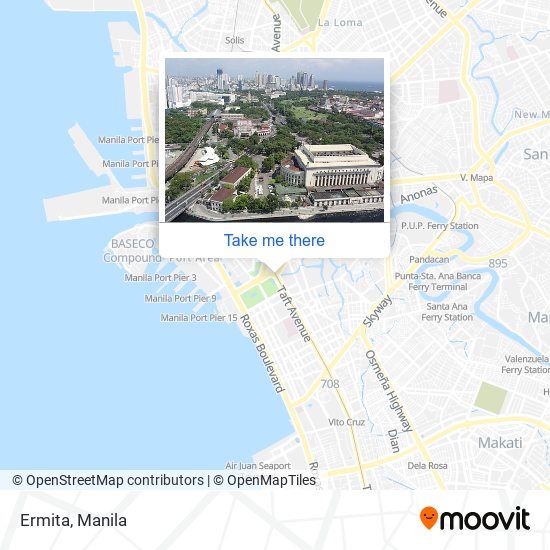Screenshot of a Navigation Map Application

This image is a detailed screenshot from a map application or website designed to help users navigate to specific destinations. The main portion of the screen features a detailed map of an urban area, with various streets and landmarks prominently displayed. At the center, there's a distinctive pop-out window showcasing a photo of a grand, large white building with a striking skyline in the background. The pop-out also features the text "Take me there," formatted as clickable hyperlinks, indicating that users can click to receive directions to this location.

At the bottom of the screen, there is a logo for the application, named "Moovid" (spelled M-O-O-V-I-D), accompanied by a cheerful, smiling location pin symbolizing the service's branding. Located in the bottom left corner of the screenshot is the text "Ermita, Manila," pinpointing the neighborhood within the city of Manila in the Philippines.

This screenshot suggests that a user has searched for a particular building or location in Ermita, Manila, and the app provides an intuitive way to navigate to this place from their current location.